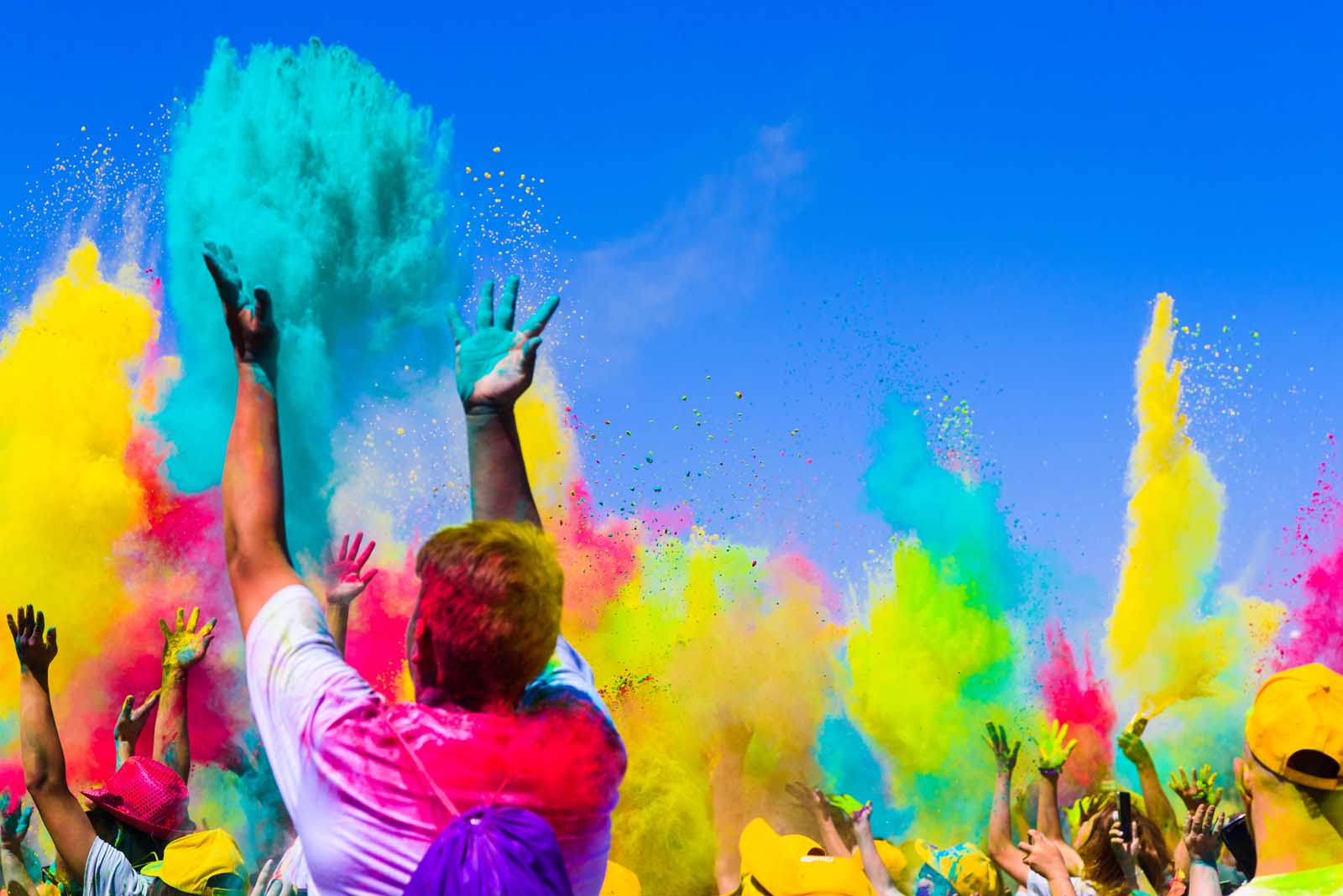In this vibrant photograph, a group of people is enthusiastically celebrating by tossing vividly colored powders into the air. Their heads and upper bodies are covered in hues of yellow, pink, red, green, and blue. Most of them wear caps, adding to the festive mood. Their hands, also smeared with colored powder, are raised in the air, capturing a dynamic moment of joy. The colorful powders create a stunning contrast against the bright blue sky. Despite the celebration's chaotic energy, certain details stand out: a person in the foreground wears a tie-dyed shirt with a white background, while another person to the right sports a yellow hat. The image, rectangular in shape, captures this lively scene with sharp detail, showing even some clumps of powder suspended in mid-air. The people appear to be facing slightly to the left, indicating their collective action towards that direction, adding depth to the photo.